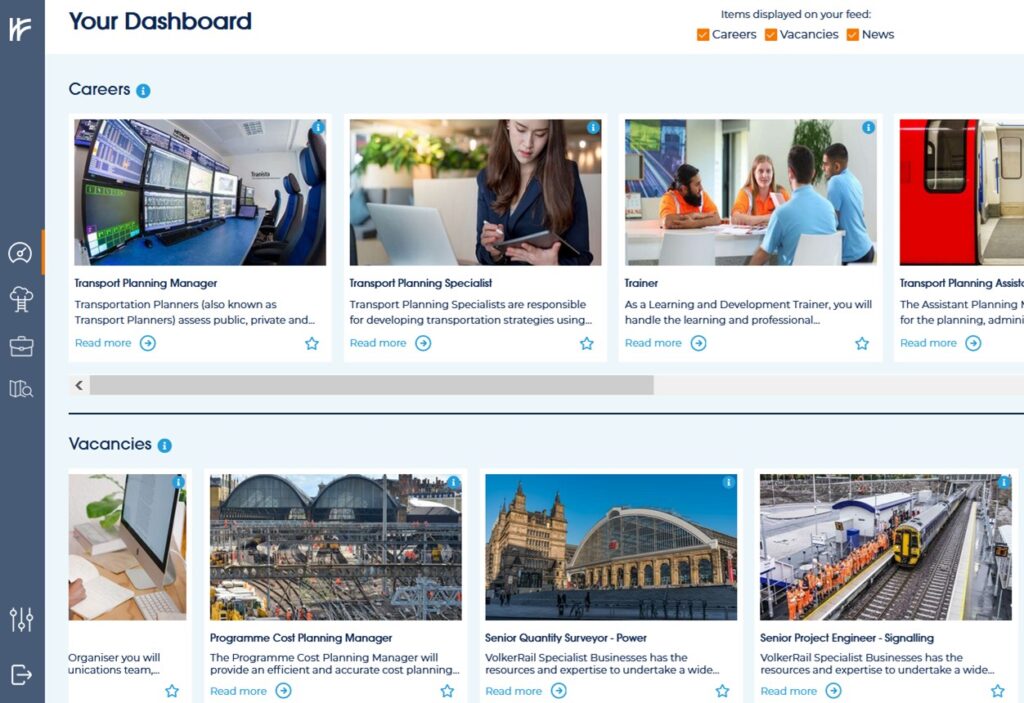This image is a detailed screenshot from a computer interface, prominently labeled "Your Dashboard" at the upper left. Just below, there's a section titled "Careers" displaying various job listings organized in a grid with accompanying images and text descriptions.

### First Row of Images and Titles:

1. **Transport Planning Manager**:
   - The image depicts a room filled with multiple computer screens positioned on desks, with a row of chairs arranged in front. The text beneath briefly describes the role: "Transportation planners, also known as transport planners, assess public, private and..."
   
2. **Transport Planning Specialist**:
   - A woman with long dark hair is looking at an iPad, with a computer positioned to her left on the desk. The description reads: "Transport planning specialists are responsible for developing transportation strategies using..."
   
3. **Trainer**:
   - The photograph shows a group discussion with four people seated at a table, two of them wearing orange shirts and the other two in blue. The caption describes the role: "As a learning and development trainer, you will handle the learning and professional..."
   
4. **Transport Planning Assistant**:
   - The accompanying image features a subway door, either blue or red. The title is partially visible, and it reads: "Transport planning assist..." 

### Second Row of Images and Titles:

This row of images and job titles appears under the heading "Vacancies."

1. **Image Partially Cut-Off**:
   - The leftmost image is slightly truncated, depicting an individual seated at a desk with a computer.

2. **Program Cost Planning Manager**:
   - The image shows an unusual building, possibly characterized by its unique architecture.

3. **Senior Quality Surveyor - Power**:
   - This picture features an old building with an arched ceiling.

4. **Senior Project Engineer – Signaling**:
   - The final image captures a train station, with a train on the tracks and a row of individuals in orange uniforms standing along the left side.

Overall, the dashboard illustrates a variety of career opportunities within the transportation and infrastructure sectors, offering visual cues and brief role descriptions to aid prospective applicants in understanding the available positions.